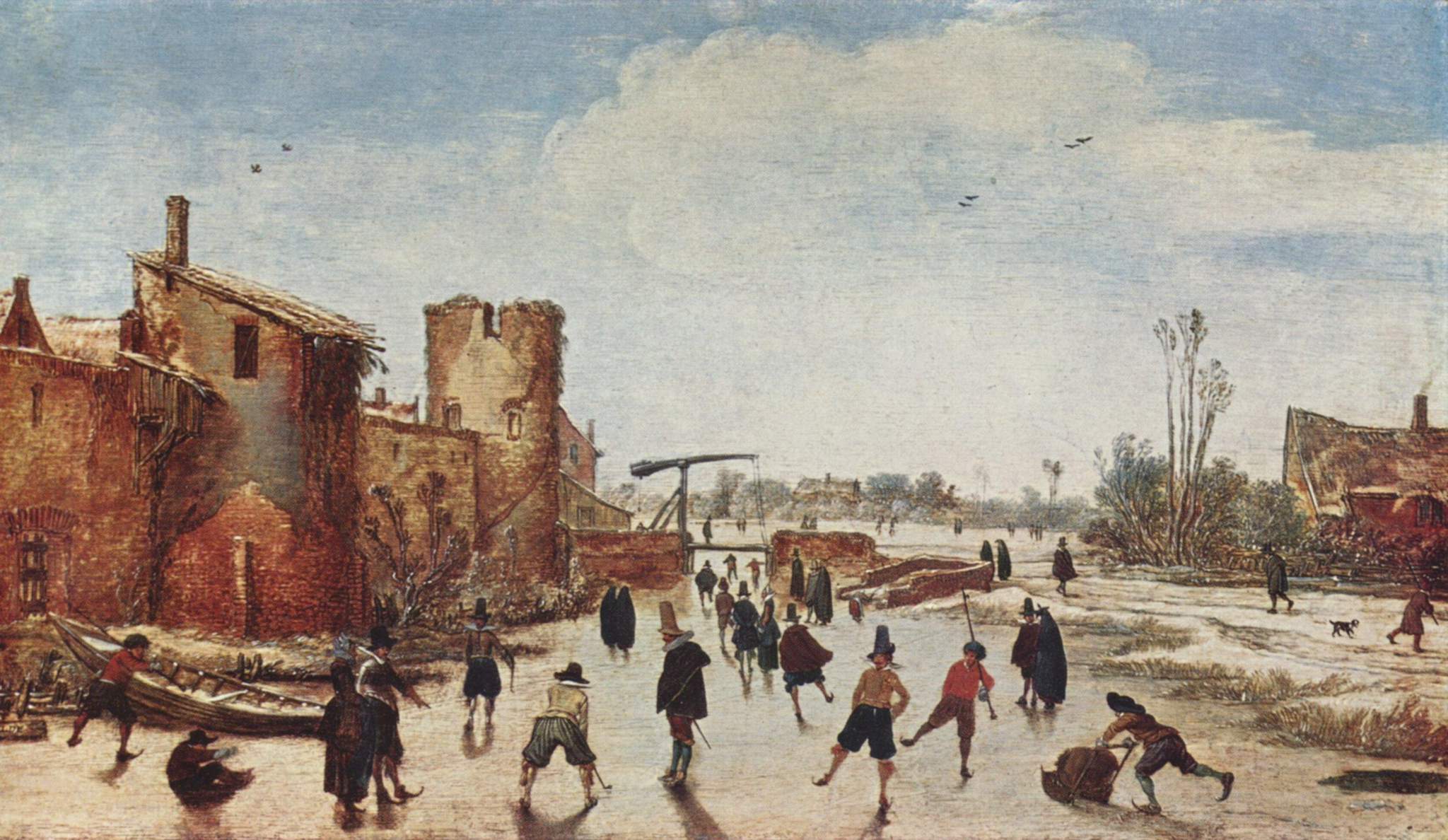This detailed oil painting features an open street scene bustling with people, set against a backdrop of aging buildings. Central to the image is a man in a top hat and light-colored shirt, paired with dark blue jeans. He stands prominently with one foot flat on the ground and the other mid-step. To his left, another man, also in a top hat, wears a yellow shirt and distinctive black-and-yellow striped pants, clutching a stick in front of him as he hunches over. Surrounding these figures are various individuals dressed in darker tones like reds, browns, tans, and blacks, some appearing to skate or move fluidly, almost as if on ice, with curved-toe shoes hinting at this movement.

The left side of the image showcases old buildings in varying states of disrepair. One structure has a sloped roof and is partially brick with bricks falling apart, revealing a weathered, steel-like frame beneath, and long fibers hanging underneath it. Another building further down has a flat top with a notch in the center and appears to have grass growing on its roof. The far right side displays a building with an arched roof and a chimney emitting smoke, set against a large tree with upward-splitting branches. In front of this building, a waterfront scene is hinted at, with a boat leaning against a bank.

The sky transitions from blue at the top to a mix of white and gray clouds, populated with birds in the upper right. The middle of the scene features a distinct, glowing street that appears wet, ending at a stand with a pole and lever, alongside hanging cables and a counterweight. This evocative painting depicts an older time, embodying the rustic charm and dynamic life of its setting.